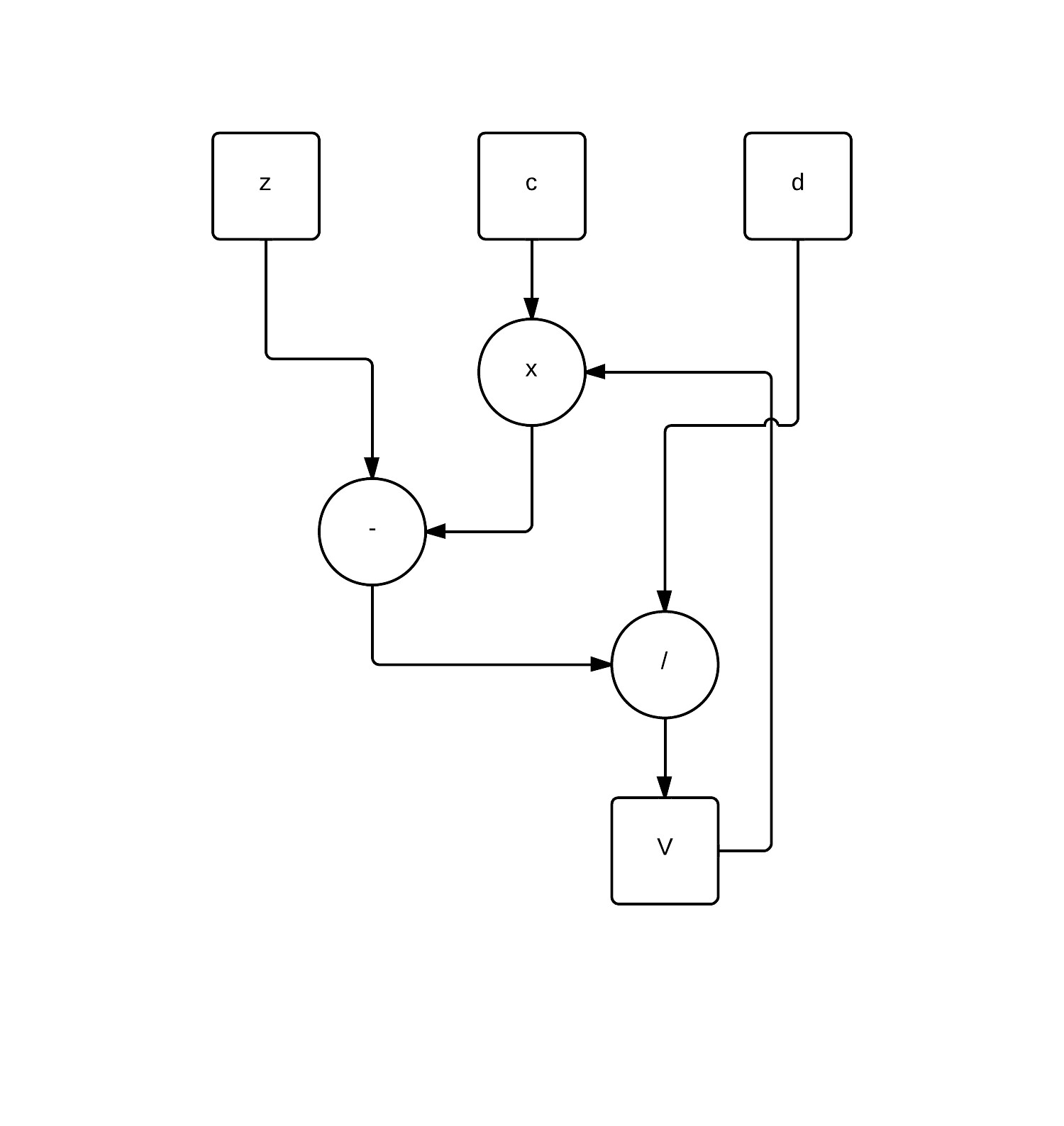A computer-generated schematic drawing is depicted, featuring a network of labeled squares and circles interconnected by arrows. At the top, three square boxes are labeled with the lowercase letters 'z,' 'c,' and 'd.'

- The 'z' box has an arrow extending downward, veering to the right at a 90-degree angle before pointing downward again, leading to a circle with a minus sign (−) in the center. From this circle, an arrow continues downward and turns right at another 90-degree angle, ending at a circle labeled 'l'. An arrow proceeds straight down from this circle to a square marked with an uppercase 'V'.

- The 'c' box in the middle has a direct arrow pointing downwards to a circle labeled 'x'. This circle connects via an arrow that moves downward and turns left at a 90-degree angle, joining the circle containing the minus sign (−). 

- To the right, the 'd' box has an arrow that moves straight down, turns left at a 90-degree angle, and continues downward to connect with the circle labeled 'l'. From this circle, another arrow descends to the square labeled 'V'.

Lastly, an arrow from the 'V' box extends rightward, ascends at a 90-degree angle, and then turns left at another 90-degree angle to loop back to the circle labeled 'x', completing the intricate schematic network.